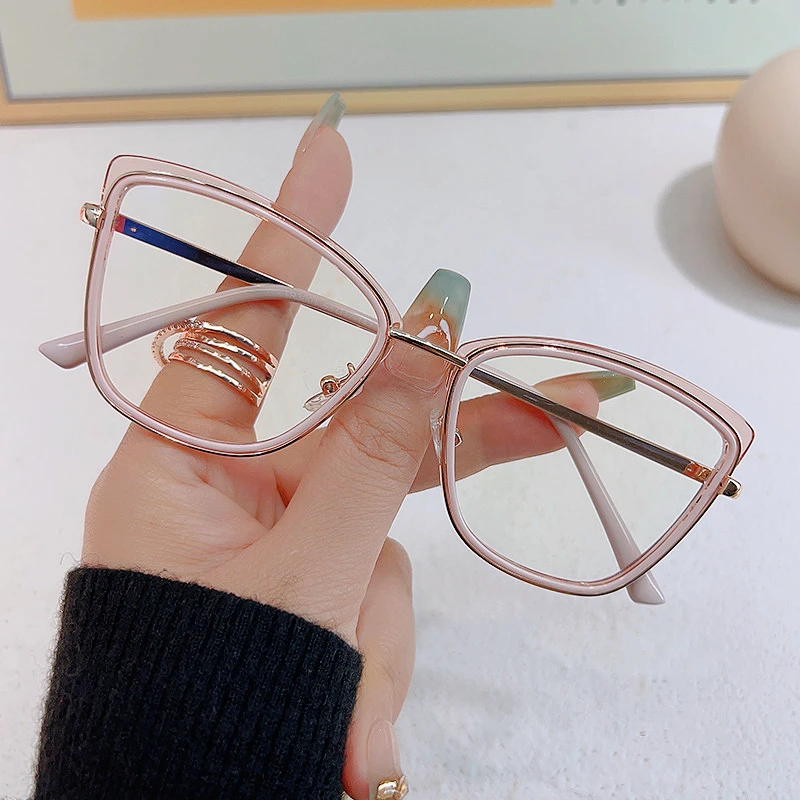In the image, a woman is holding a pair of square-shaped glasses with a translucent pink frame and copper-silver metallic rims. Her hand, adorned with multiple rings and sporting a stylish acrylic manicure with teal and clear marble design, is extended against a white table surface. She wears a black-sleeved shirt that reaches her wrist. The background features a beige lamp casting a shadow, and the partial edge of a framed piece of art, which is not fully in view. The entire scene emphasizes the contrast between the elegance of her manicured hand and the simplistic background.